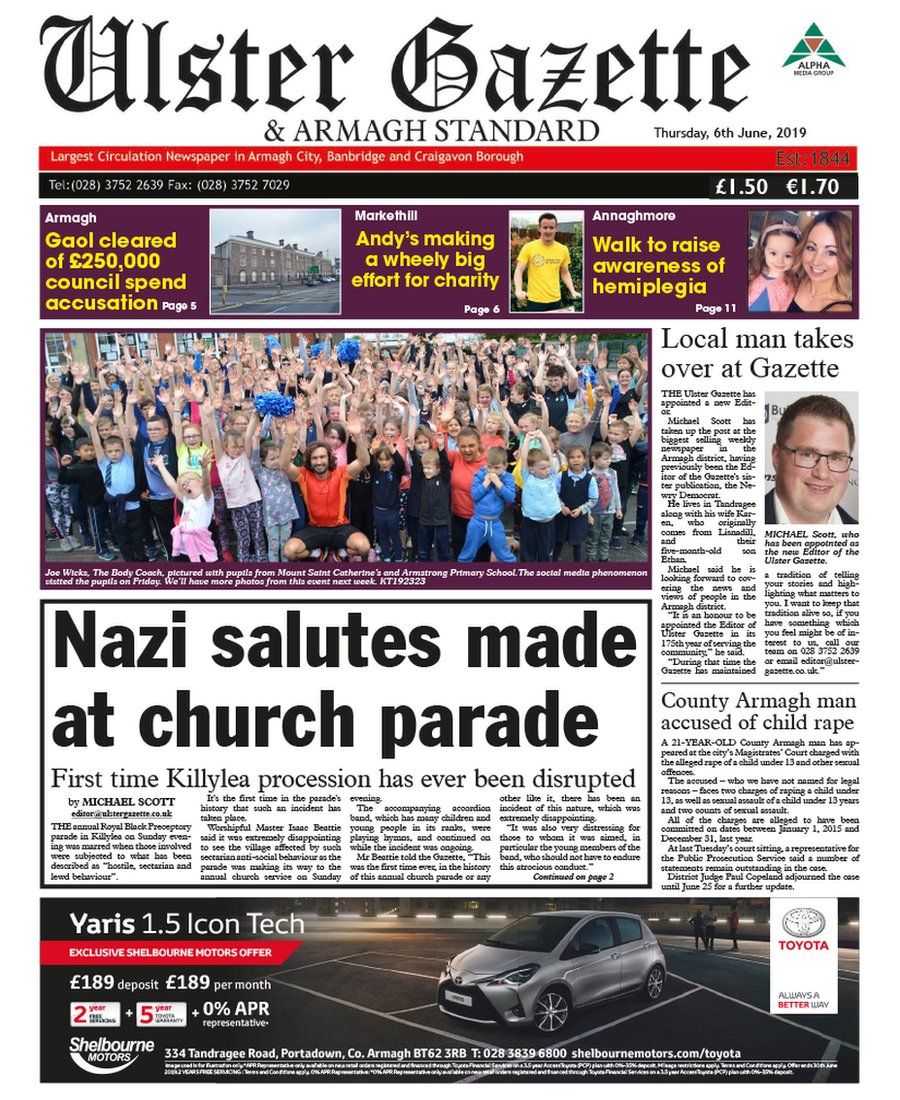The front page of the Western Gazette, dated Thursday, 6th June 2019, features a blend of local news and community highlights. At the top, the publication name "Western Gazette" is prominently displayed, although "Gazette" is misspelled as "GEASETTE." The masthead also includes "ARMAGH Standard" and the publication date. 

In the top right-hand corner, there's a distinctive logo comprising a green triangle with a brown triangle in the center. Encircling these triangles is a white space with the text "ALPHA" in all caps, followed by "media group" centered below it in black letters.

Below the logo, the headlines capture immediate attention. On the far right, against a purple background, one headline reads: "ARMAGH goal cleared of £250,000 council spend accusation." Next to it, an image features a man in a white shirt and black pants with short brown hair. This piece is titled "MARKETHIL" in yellow, featuring the caption, "Andy making a willy big effort for charity."

Adjacent to this is another image of a woman with shoulder-length dirty blonde hair wearing a strapped black dress. She is holding a child with hair bows, dressed in a pink dress over a blue undershirt. The headline, "ANNAGHMOR," is in white text, followed by the yellow text, "Walk to raise awareness of hemiplegia."

To the left of the page, a group of people are depicted under the headline, "Nazi salutes made at church parade." Completing the news feed on the right side, another headline reads, "Local man takes over Gazette."